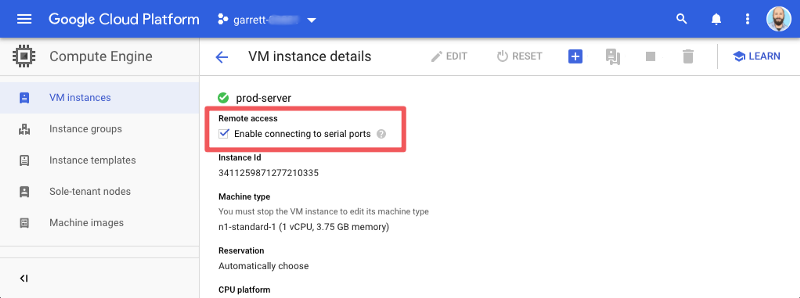The screenshot depicts an application interface from Google Cloud Platform. The top section of the image features a blue bar. On the left side of this bar, a menu is partially visible. To the right of the "Google Cloud Platform" label, there's a triple circle logo accompanied by the name "Garrett Dot," which is blurred out in a dropdown menu. Continuing to the right, the bar includes a search bar, a notification bell, an icon with three vertical dots, and a profile picture represented by a cartoon image of a bald man.

Below this top bar, on the left side, there is a sidebar menu under a heading called "Compute Engine". This sidebar contains several categories: 
1. VM Instances
2. Instance Groups
3. Instance Templates
4. Sole Tenant Nodes
5. Machine Images.

On the right side of the screen, there is a section titled "VM Instance Details," indicating that the interface is currently within the VM Instances category. This section contains several function buttons: Edit, Reset, a plus button (presumably for adding a new instance), a bookmark button, a pause button, a delete button, and a blue "Learn" option.

Beneath these buttons, there's a checklist item labeled "Prod Server" with a checkmark indicating that remote access has been enabled along with a note about connecting to serial ports. This section is highlighted by a red border. Further down, detailed instance information is provided, including an Instance ID composed of a long sequence of at least 15 digits, the Machine Type labeled as "N1-Standard-1" which specifies 1 V CPU and 3.75 GB memory, Reservations configured to "automatically choose", and the CPU Platform details.

Overall, the screenshot provides a detailed view of Google Cloud Platform's Compute Engine section, specifically focusing on the VM Instance Details and associated functionalities and settings.